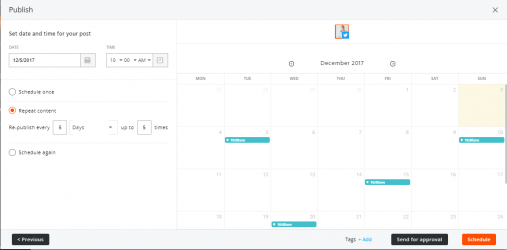This is a somewhat blurry screenshot of a settings and Calendar app interface. At the top, there is a gray navigation bar stretching across the width of the screen. On the left side of this bar, the word "Publish" is displayed in black font, while an "X" icon to close the menu is located at the far right.

Below the gray bar, the screen features a white section. In the upper left corner of this section, the text "Set date and time for your post" is prominently displayed. Below this, there are two input fields for specifying the date and time. The date field is populated with "12/5/2017," and the time field shows "10 a.m."

Further down, there are multiple selectable options in a list format. The first option is a small clickable circle labeled "Schedule Once." The next option is another clickable circle labeled "Repeat Content," which has been selected. Directly below this selection, the text "Republish every six days up to six times" is visible. There is also another circle, which is not selected, labeled "Schedule Again."

To the right of the white section is an open calendar view for December 2017. The calendar contains squares representing the days of the month, arranged in a grid labeled from Monday through Sunday. There are several entries in the calendar, but they are too small to read clearly.